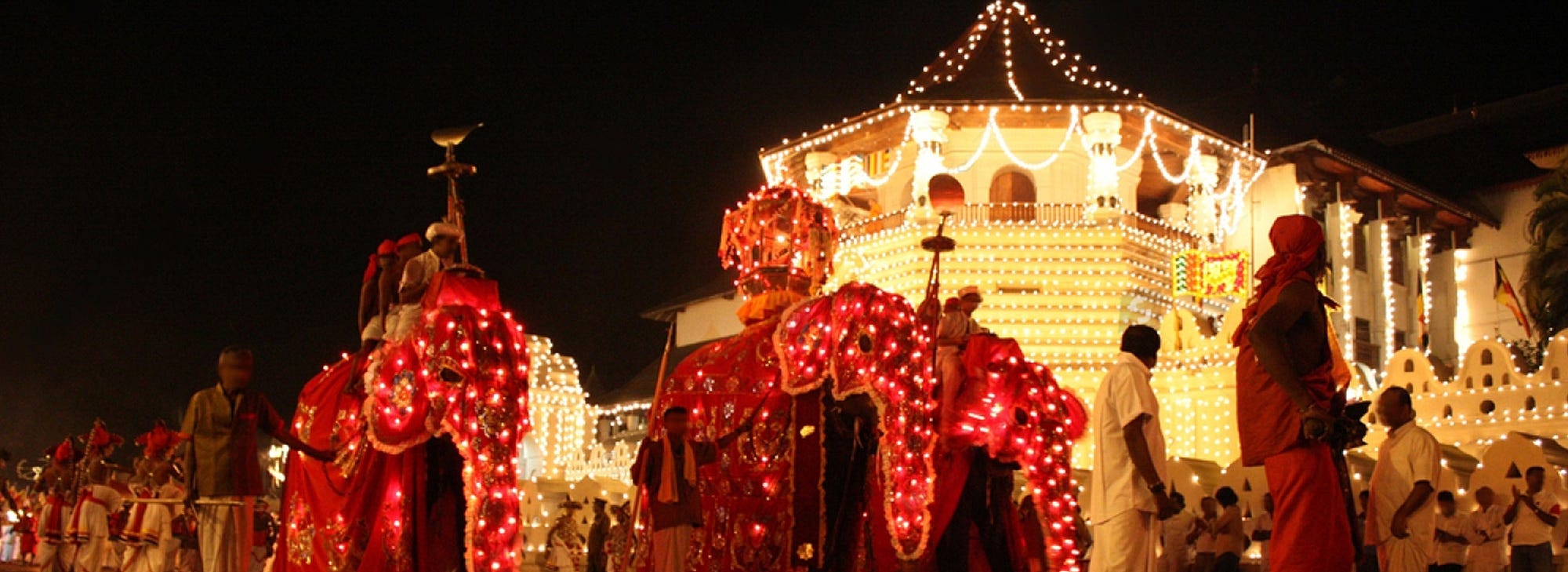The image depicts a vibrant nighttime celebration set against a pitch-black sky, prominently featuring a grand, multi-sided building illuminated with hundreds of white lights forming intricate, triangular patterns on its roof. This beautifully lit structure, which resembles a large temple or an ornate pavilion, stands as the centerpiece with its white pillars framing an open balcony that overlooks the festivities below.

In the foreground, a lively parade unfolds, characterized by a mix of cultural and traditional elements. A notable highlight is the presence of three elephants, adorned with red glowing lights and elaborate red carpets draped across their backs. The elephants' faces are covered with illuminated decorations, giving them an otherworldly, glowing red appearance while their eyes peek through the coverings. 

Surrounding the elephants are numerous people, many dressed in traditional Indian attire. Some hold the elephants in line, while others march in celebration, creating a dynamic and festive atmosphere. In the background, men in white outfits and palm trees add depth to the scene, suggesting a locale in a desert region. The air is filled with an infectious sense of joy, as people clap, move about, and immerse themselves in the ongoing celebration.